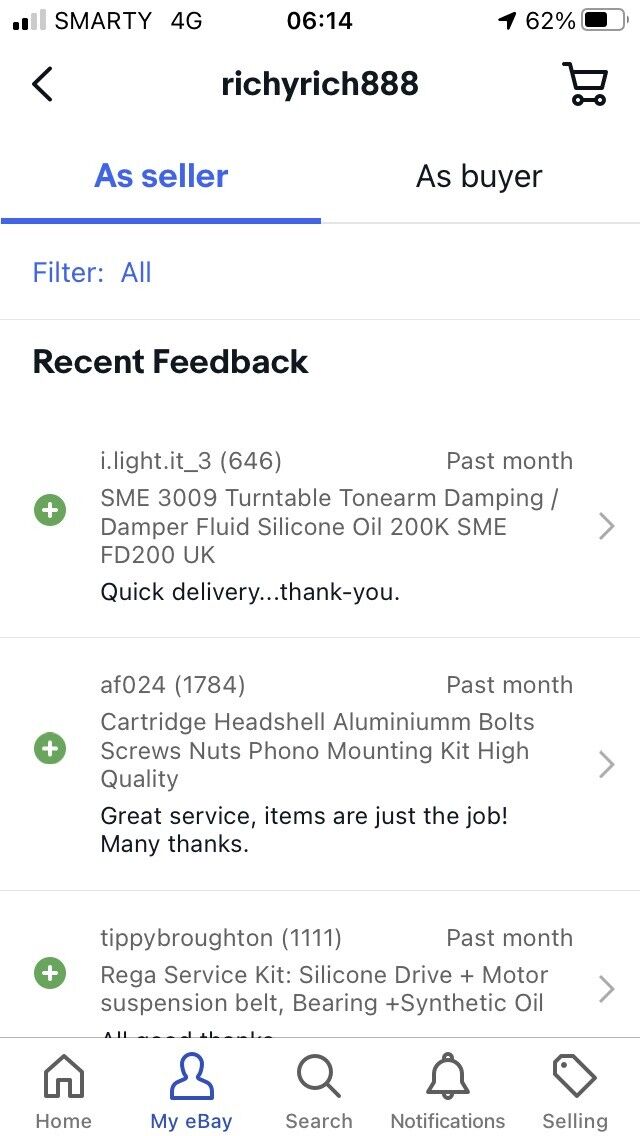This image, captured from a cell phone screen, prominently displays the user interface of an app. At the top of the screen, the name "Richie Rich 888" is visible. To the right, there is an icon of an empty cart, suggesting a shopping feature. On the far left, a left-pointing arrow indicates a back navigation option.

The status bar at the top reveals various details: the network provider is labeled as "Smarty," with a signal strength of "4G". The current time is displayed as 06:14. The battery life is shown at 62%, accompanied by a battery icon.

Towards the lower section of the screen, navigation options include "Filter," with the choices displayed as "alt" or "all," and a section titled "Recent Feedback." This area features three green circles, each containing a white plus sign. Underneath the recent feedback header, there is an item labeled "I light it," followed by the description "cartridge head shell aluminum bolts." Below this, the username "tippy Broughton 1111" is shown, likely indicating the user who provided the feedback or item details.